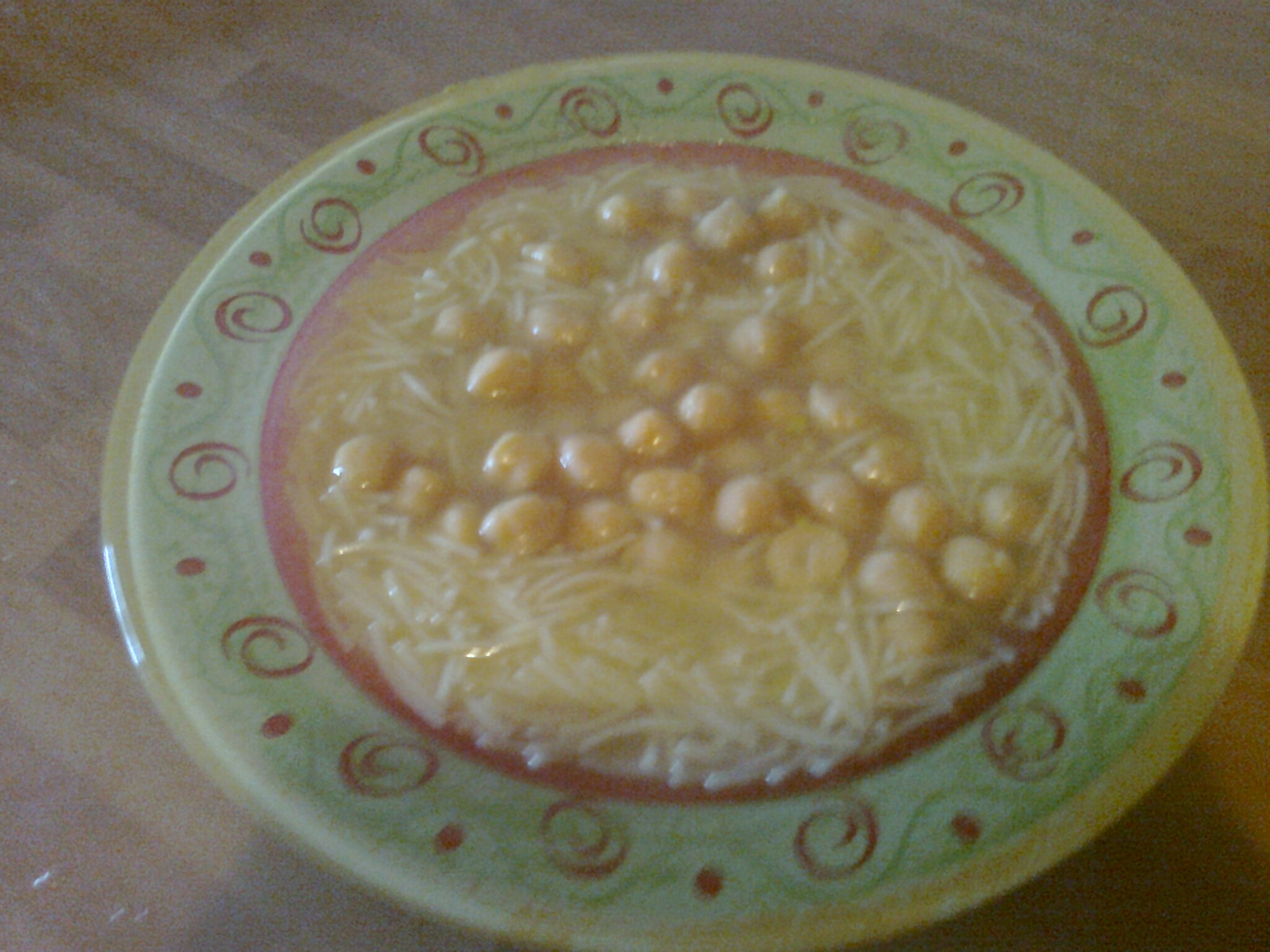This is a blurry photograph of a bowl of noodle soup with chickpeas, resting on a wooden table. The round bowl features a light greenish-blue color with faint, intermittent swirls and stripes. Marine-colored swirls in a 'G' shape or '@' symbol pattern grace the bowl, interspersed with maroon dots and curls that repeat around its circumference. Inside the bowl, thin, small white noodles and tan, round chickpeas float through the soup.